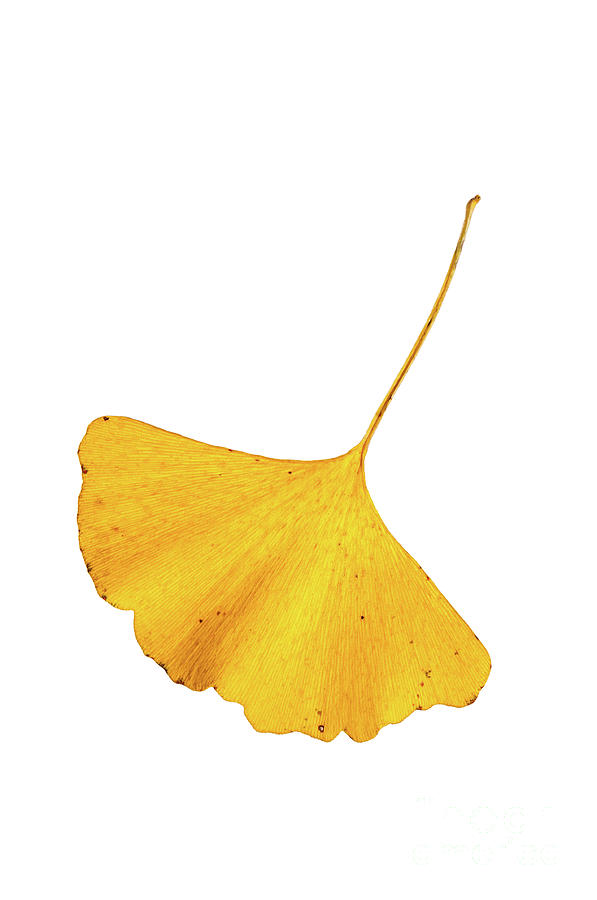In this meticulously crafted, seemingly photoshopped image set against a stark white background, a single, delicate leaf graces the frame. The leaf is anchored by an extremely narrow stem, which extends diagonally from the upper right corner, drawing the eye downward. This slender stem blooms into a fan-shaped leaf, positioned diagonally from the upper left to the lower right of the image. The leaf, a rich golden yellow, features intricate waves and ridges along its edges, lending it a textured and naturalistic appearance. Streaks of brown subtly shade the leaf, suggesting a touch of discolouration or the natural aging process. The tips of the leaf also display specks of brown, further enhancing its lifelike quality.